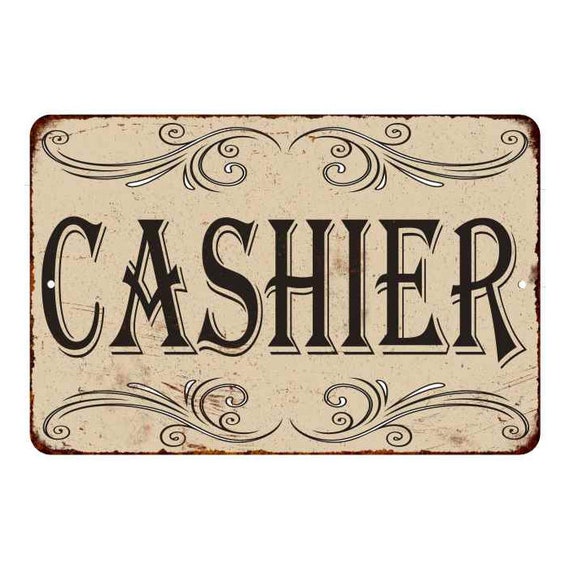The image displays a rectangular, old-style sign with rounded edges and overall dimensions of a square. The sign features a worn, rustic appearance with a background in a light tan or pale yellow hue, showing signs of rust and wear along the borders and corners. Central to the design is the word "CASHIER," prominently displayed in large, black, all-capital letters with a clear outline and shadow effects that lend a 3D appearance. Above and below this text is decorative scrollwork composed of intricate curls and spirals, more detailed at the bottom than at the top. The scrollwork on both edges mirrors each other, with three smaller spirals and one larger spiral. Additionally, visible in the center left and center right of the sign are small holes likely meant for hanging the sign.